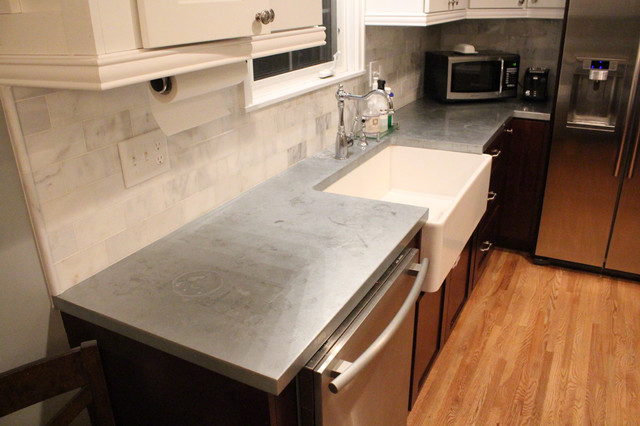This image portrays a clean and modern kitchen with an isometric view. The kitchen features a large white basin sink situated in the middle of a gray concrete countertop, which is completely free of clutter except for a microwave, a toaster, and some cleaning supplies. On the right side of the counter, there is a stainless steel refrigerator equipped with a water spout and ice maker on the left door. Below the counter, on the left side, resides an upscale, stainless steel Bosch dishwasher. The drawers and cabinets below the counter vary in color, with brown drawers and cabinets under the sink, and additional storage to the right of the sink in the form of brown cabinets. 

The backsplash consists of white and gray marble tiles, complemented by two light switches and two electrical outlets on the left wall panel. Above the countertop are white cabinets with silver handles, one of which has a paper towel roll hanging beneath it. A window is placed directly above the sink, allowing natural light to illuminate the room. The wooden floor, in shades of brown and dark brown, contrasts with the clean, gray tones of the countertop and appliances, enhancing the kitchen’s warm yet contemporary feel.